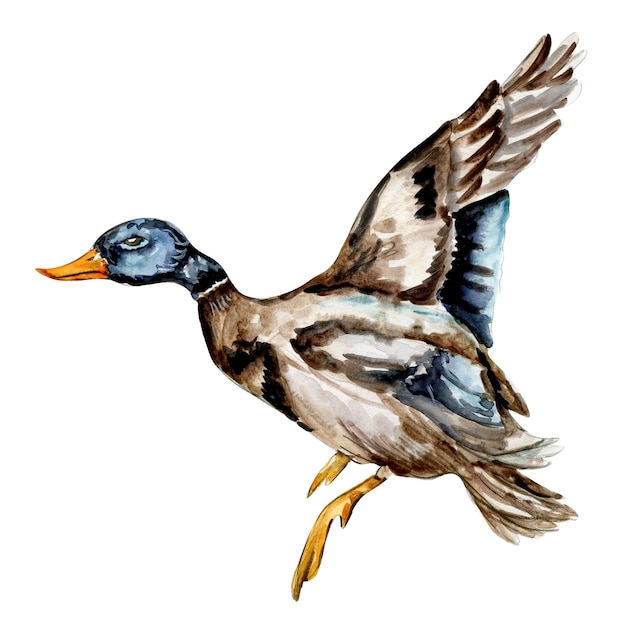This detailed illustration captures a mallard duck in flight against a white background, moving from right to left, as if it has just taken off from the water. The duck, depicted in a side view, has an elongated orange bill and a blueish-gray head adorned with black swirls. Its almond-shaped black eyes add a sense of focus as it gazes into the distance. The neck transitions from blue to a ring of white feathers, seamlessly leading into a body that showcases a mix of brown, white, and tan hues.

The wings, extended and raised upward, reveal detailed brown-tipped feathers and a small patch of blue near the body. A square of blue is visible on the lower part of the duck's body near the wings. The tail feathers, predominantly brown with hints of white, fan out behind it. Below, the duck’s light orange feet dangle, with the left foot more prominently extended.

This watercolor or possibly acrylic painting, rich in detail, appears poised between realism and artistic illustration, making it suitable for a nature-themed book or an ornithological guide.